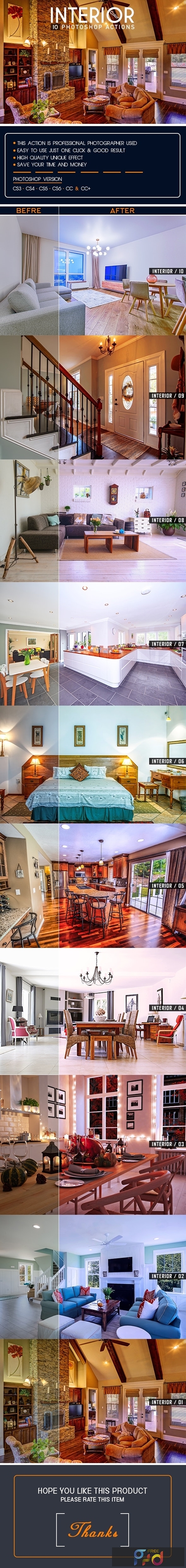The image displays a poorly designed, horizontally stretched website advertisement, making the texts and images difficult to read and visually unappealing. At the top, in a large font, the word "INTERIOR" stands prominently. Below this, the headline reads "10 Photoshop Actions." Additionally, there is some white text stating that these actions are used by professional photographers, are easy to use with just one click, and produce good results. It also mentions that these actions save time and money, though the exact quality of the results is questionable. The advertisement specifies compatibility with Photoshop versions CS3 through CS6. The central part of the image is cluttered with numerous photos that are also stretched horizontally, detracting from their quality. At the bottom, there's a message asking viewers to rate the product and expressing hope that users will like it, ending with a polite "thanks."